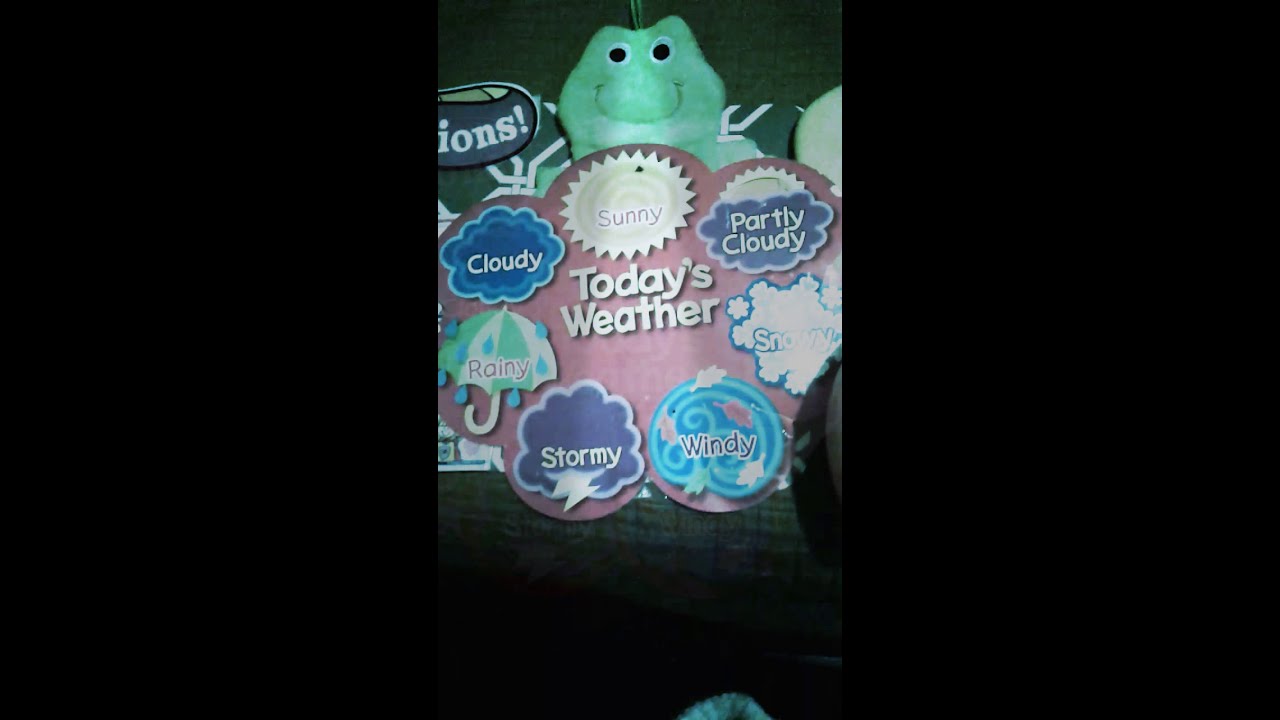A horizontally aligned rectangular image features the face of a green toy frog, resembling Bang Lee the cartoon character, with a U-shaped mouth and large black-and-white eyes. In front of the frog is a cloud-shaped cardboard sign with a red background and the words "Today's Weather" in white print at the center. Surrounding this text are various weather icons arranged in a circular pattern: a yellow sun labeled "sunny," a partly cloudy symbol with a sun partially obscured by a cloud, a gray cloud labeled "cloudy," a blue snowflake indicating "snowy," swirling lines with leaves for "windy," a gray cloud with a lightning bolt for "stormy," and a green-and-white umbrella with blue raindrops for "rainy." The palette, shaped like a flower, appears to be a teaching tool designed to educate children about different weather conditions.